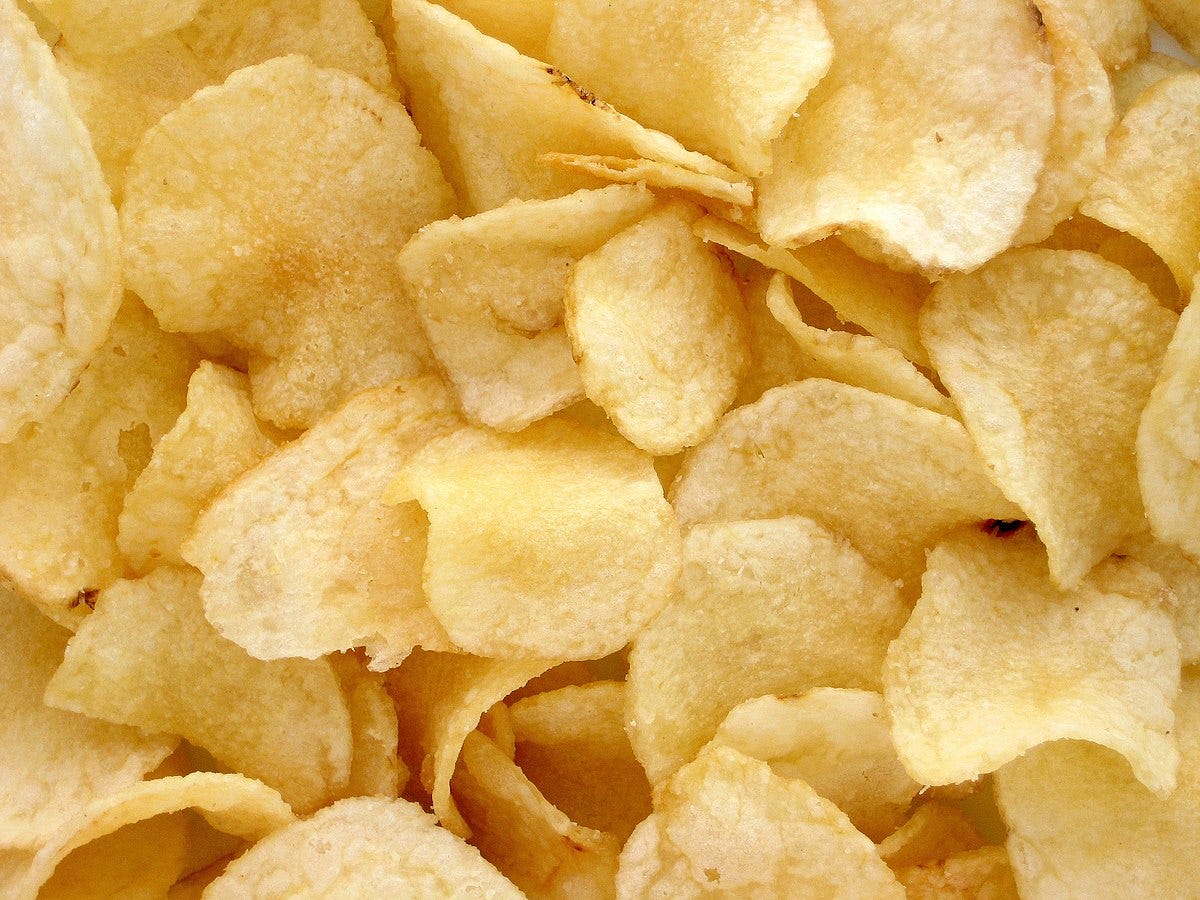This photograph features a tightly framed, close-up view of a pile of golden yellow, thick-cut potato chips scattered from one edge of the image to the other. Unadorned by bowls or bags, the crunchy snacks fill the frame entirely, their appetizing texture and color illuminated by clear, bright lighting. The chips vary in shape and size, some resembling round discs while others curve like little saddles. Touches of brown or red at the edges suggest a homemade quality, with visible hints of potato skin and occasional small holes adding to their crispy allure. The uniform appearance and slightly thicker cut hint at a kettle-cooked style, complete with a light sprinkling of salt around the edges. With no other objects or branding present, the focus remains solely on the enticing pile of potato chips.